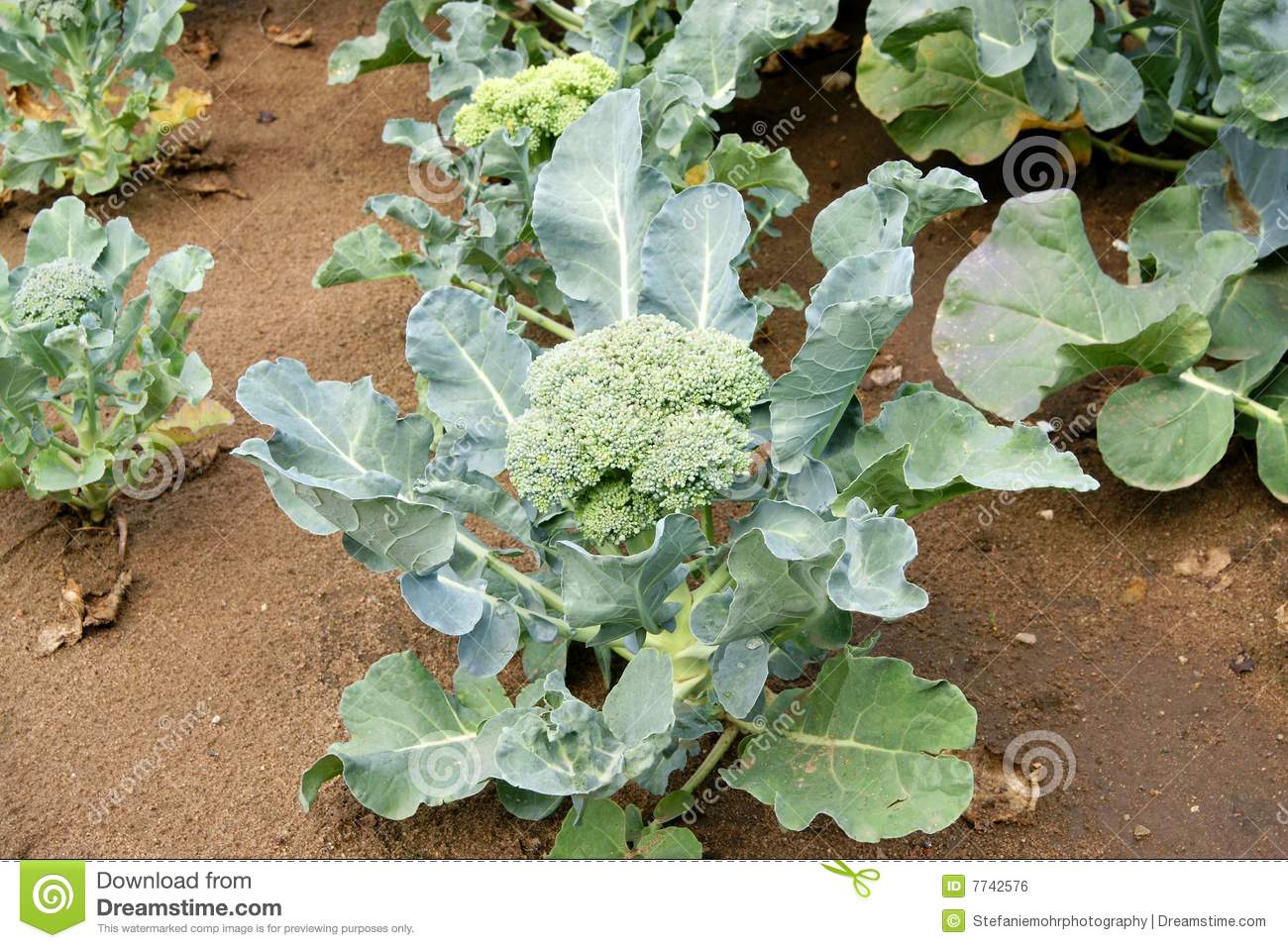The image displays a collection of plants growing in firm, brown soil that varies in wetness, giving the ground a dark, patchy appearance. The plants, which resemble broccoli, have multiple large leaves extending from their stems in various angles, creating a lush and leafy display. Central to each plant is a flowery cluster that resembles the top part of broccoli. The plants are in different stages of growth, evidenced by their varying sizes and the faded, washed-out greens of some leaves. The overall scene has a dense and detailed natural texture, with occasional small specks and rocks dotting the soil. Overlaying the image are watermarks from Dreamstime, including white angled text and a green banner with a white swirly logo, suggesting the image is sourced from the internet.